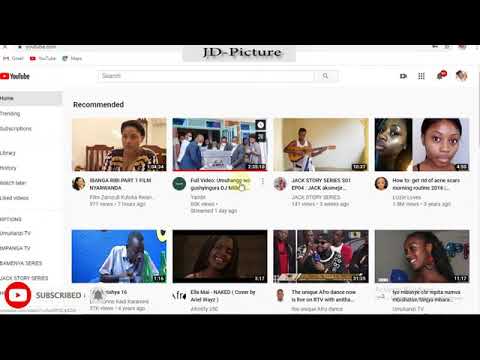A blurry screenshot of a YouTube search results page, featuring the username "JD Pictures" at the top. The search bar is empty. On the left sidebar, the menu options listed from top to bottom are: Home, two unreadable labels, Library, two more unreadable labels, Liked Videos, and five additional unreadable titles. The main content shows eight video thumbnails arranged in two rows of four. 

In the top row, from left to right: a woman sitting in a living room, a group of people in suits wearing masks, seemingly carrying a coffin out of a building, a man standing while holding a guitar, and two different images of a woman looking at the camera.

In the bottom row, from left to right: a man sitting in front of a blue screen, a woman smiling at the camera, a man talking into a microphone, and a profile view of a woman standing against a white background. The poor image quality and blurry text make most of the titles difficult to read.